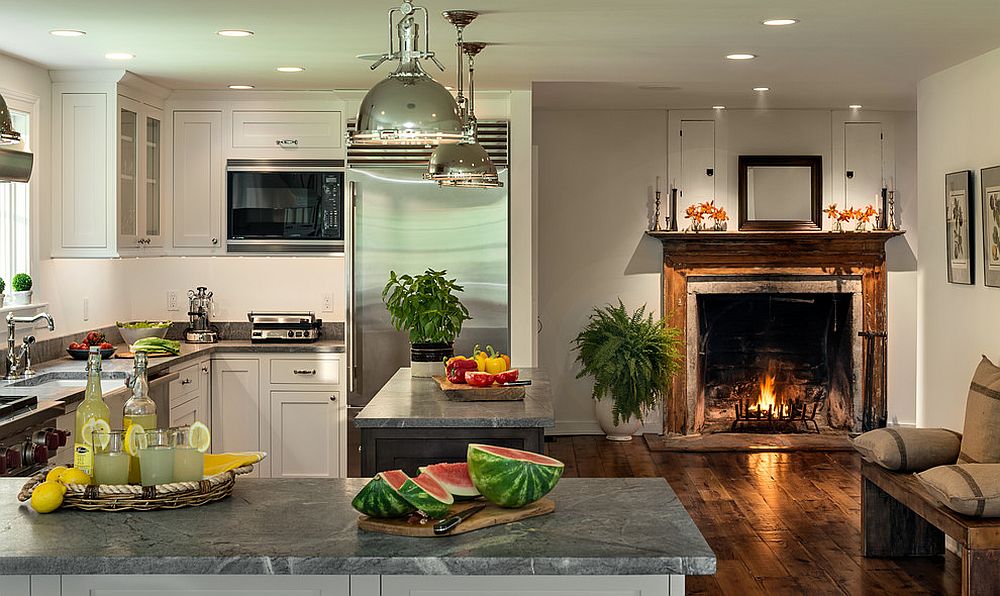This image captures a sophisticated and modern kitchen seamlessly integrated with a cozy living room area. Dominating the left side of the composition is a sleek kitchen setup, featuring gray marble countertops. On the left countertop, a cutting board displays a half watermelon and three slices alongside a sharp knife. Close by, a wicker tray adorned with bottles and glasses of lemonade, and whole lemons sits prominently. Appliances such as a microwave and a toaster oven are nestled among white cabinets with gray handles above. 

A massive gray refrigerator stands to the left, with a kitchen island positioned centrally. The island showcases an array of peppers, a potted plant, and hanging lights that add a touch of elegance. The right side transitions into a living room area characterized by a roaring fireplace beneath a mantel adorned with assorted items, and a wooden bench outfitted with plush cushions. The backdrop features stylish photographs mounted on the wall. The entire space exudes a modern and luxurious ambiance, all tied together with a warm wooden floor extending across both the kitchen and living room areas.